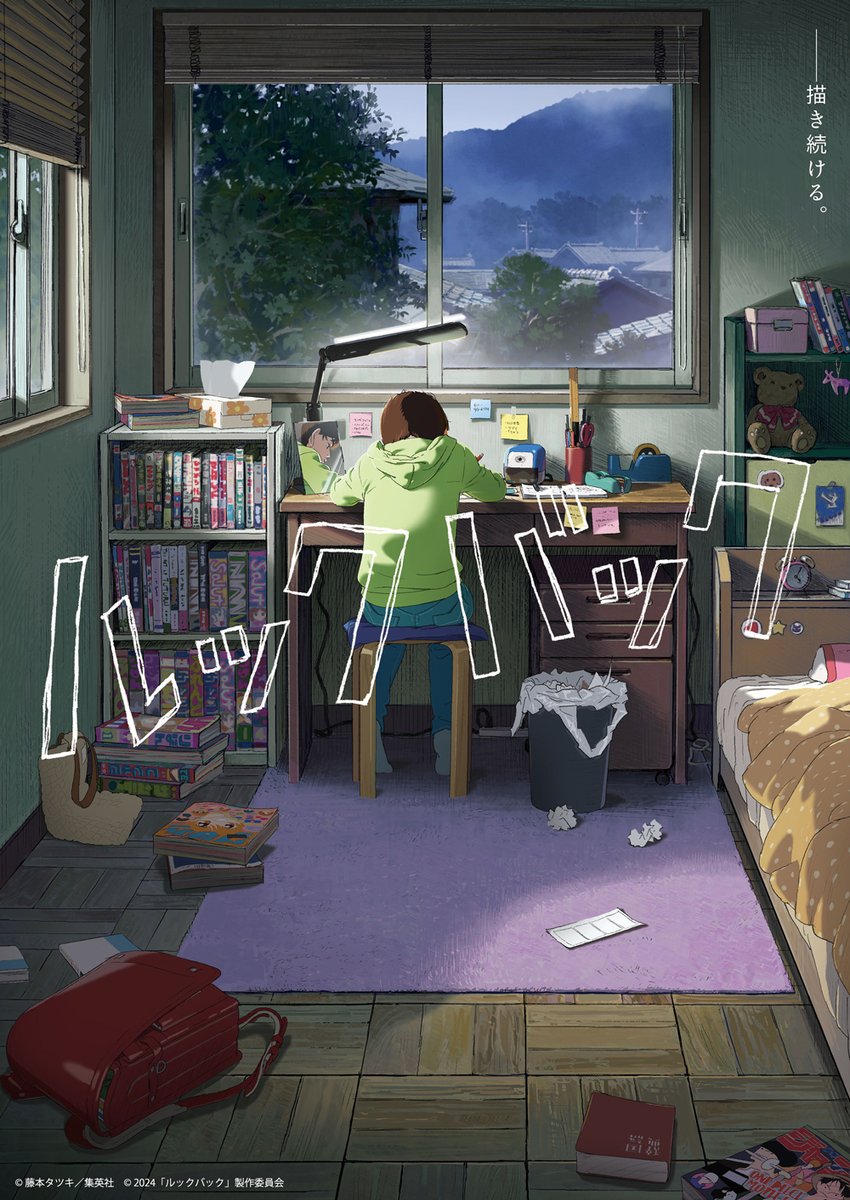The image is a detailed color illustration reflecting a serene Japanese study setting. The focus is on a student, viewed from behind, seated on a stool at a desk. The student, dressed in blue pants and a green hoodie, appears to be writing diligently. On the left side of the desk, a bright desk lamp casts light over their workspace, which is filled with various objects including a tape dispenser and a pencil cup.

In the background, a double window offers a picturesque view of lush trees and rooftops with a majestic mountain rising in the distance. Mist gently envelopes the top of the mountain, adding a sense of tranquility to the scene. The wide-slat blinds on the window are pulled up, allowing an unobstructed view of the scenery.

To the left of the desk, a short, three-shelf bookcase stands pressed against the wall. This bookcase is crammed full of books on each of its shelves, with an additional stack of books piled on the floor in front of it. A box of facial tissues and a couple more books rest on the top of the bookcase. The desk is pushed right up against this bookcase, maximizing the use of space.

The room features a parquet style floor, partly covered by a lavender purple area rug that extends under the desk and stool. Next to the desk sits a waste basket lined with a white plastic bag, filled with crumpled paper. On the right side of the desk stands a freestanding green bookcase, holding a teddy bear and a purple box on its shelves. This detail, along with the presence of a red children's backpack at the lower left side of the image, suggests the room likely belongs to a young girl.

Japanese vertical writing adorns the wall above the shelf on the left, adding a cultural touch to the setting. On the right edge of the image, the corner of a bed is barely visible, emphasizing the multifunctional use of the room. Scattered on the floor in the bottom right are more books, one of which appears to be a magazine featuring a face, possibly a fashion magazine, and a red-bound book.

White outlined, handwritten text is superimposed across the image, seemingly reading "hawa hawa." The exact significance of this text is unclear, but it adds a whimsical element to the overall illustration.